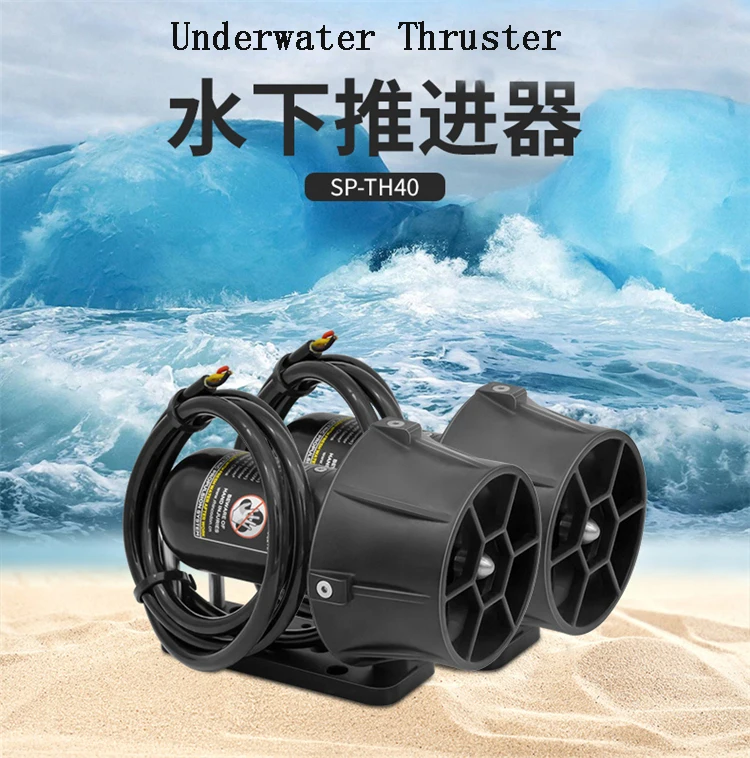In the image, there's an advertisement for a scuba diving product called an underwater thruster, with the model number SP-TH40. The setting appears to be outdoors with a beautifully photoshopped or AI-generated ocean wave rolling onto a sandy beach, extending up to a clear sky. The central focus of the image is a pair of black, gray, and white underwater thrusters. Each device features a large fan at the rear, likely around a foot and a half in diameter, and cylinders of gas at the front, connected by thick hoses ending in brass nozzles. The text "underwater thruster" appears at the top of the image, accompanied by a line of Chinese characters that reinforce the product's name. The image employs colors such as blue, light blue, yellow, red, black, gray, and white, creating a vibrant and eye-catching scene.